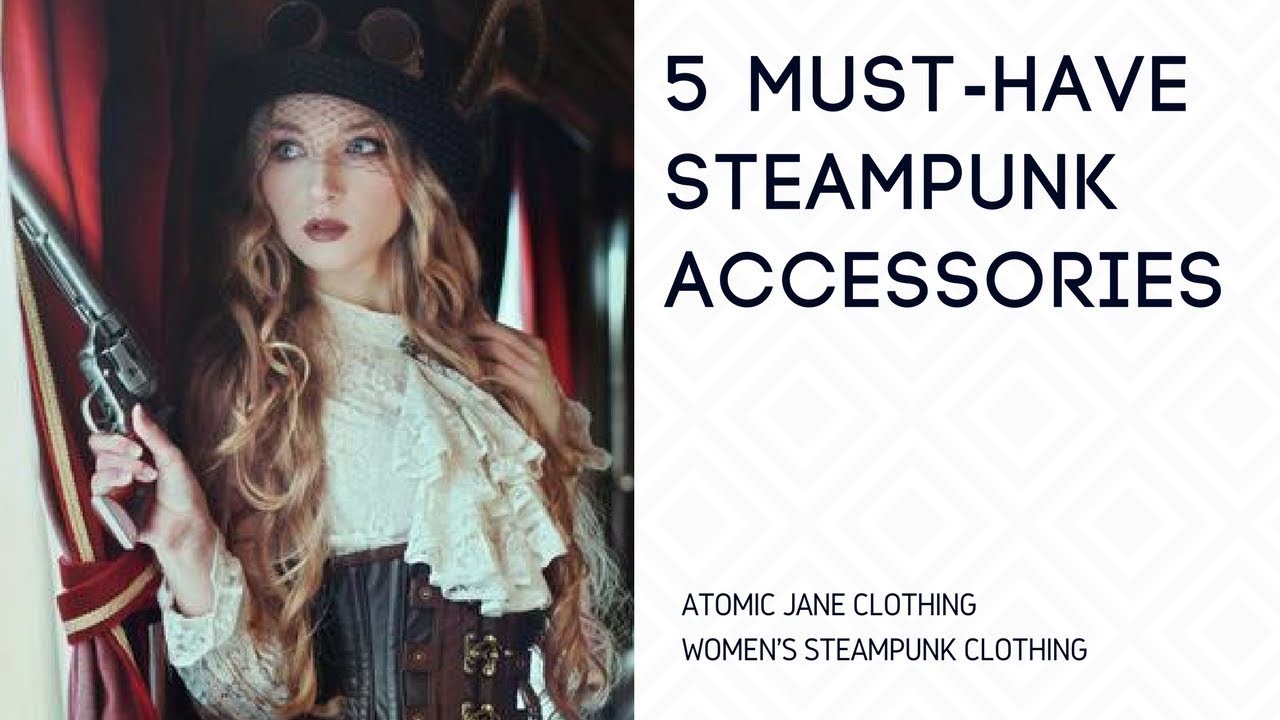The image portrays a striking steampunk-themed scene, likely an advertisement, featuring a serious-looking woman standing against a red curtain backdrop. She sports a black hat adorned with vintage goggles and has long, curly, dirty blonde hair with blue eyes and red lipstick. She wears a white, frilly lace blouse underneath an elaborate black and brown corset, accented with lace details. Her attire is completed with a pair of goggles and a black hat. The woman is holding a black revolver with a brown handle in her right hand, poised as if ready to use it.

The set design suggests a Victorian-era ambiance, with the woman positioned in a manner that implies readiness or alertness. This is enhanced by her stance and the weapon she holds. The background text reads "Five Must-Have Steampunk Accessories" in bold black letters. Below, in thinner black font, the advertisement credits "Atomic Jane Clothing" for the woman's steampunk attire. All elements of the photo come together to create a vivid and clean visual, effectively highlighting the steampunk aesthetic and the products advertised.